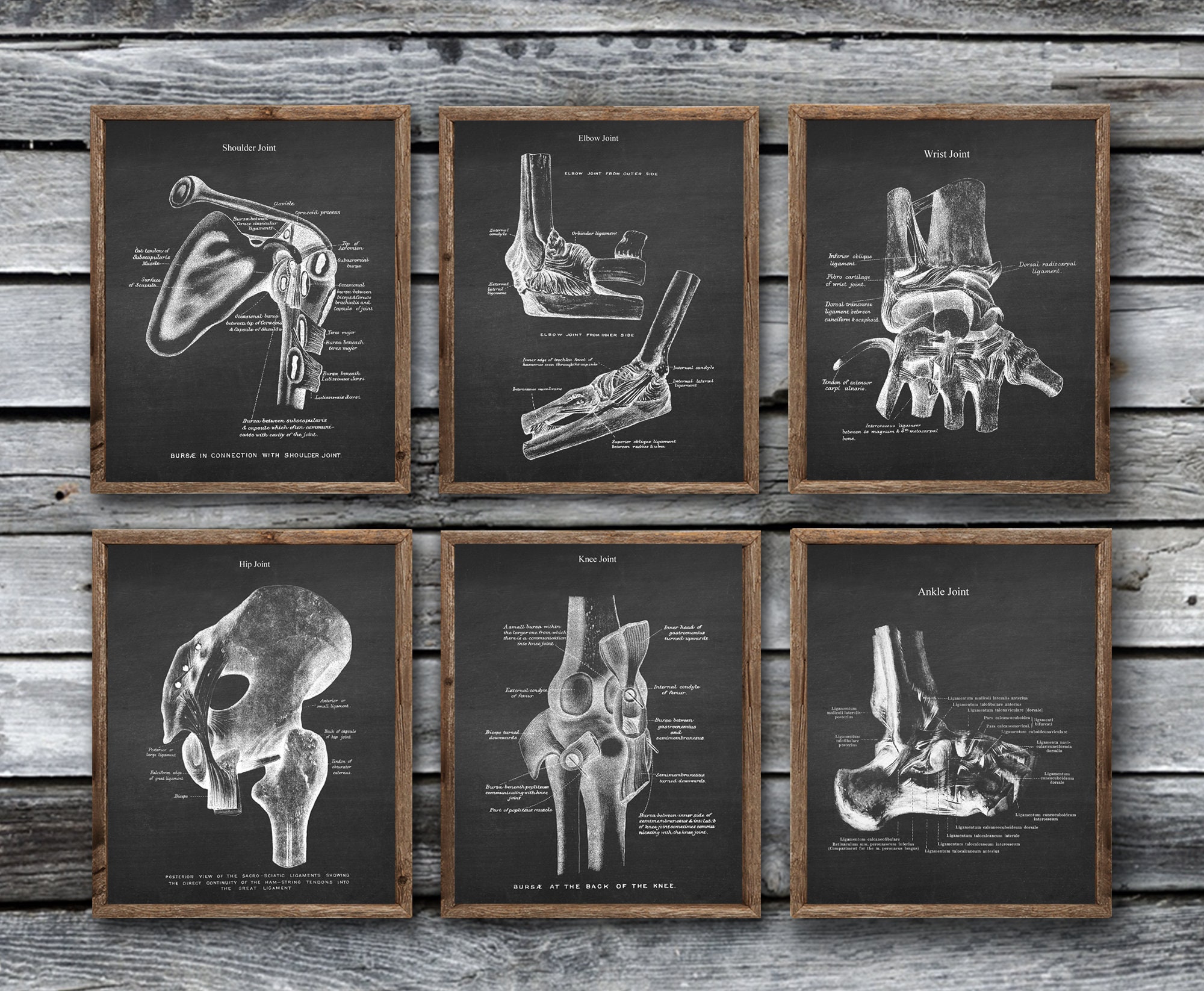The image is a full-color, square photograph that appears to be carefully staged. It features a background of an old, worn wooden wall with conspicuous slats between the boards. In the foreground, two rows of three vertically rectangular frames are prominently displayed. Each frame is identical, being made of brown wood, and encloses a black background that highlights detailed white drawings of human bones. These black-and-white images, though adorned with descriptive text, have labels too small to be read clearly.

From left to right, starting with the top row, the drawings depict the shoulder joint, elbow joint, and wrist joint. The bottom row features images of the hip joint, knee joint, and ankle joint. Each drawing meticulously points out specific bones and parts associated with these joints, providing a comprehensive view of the skeletal structure in these areas. The clear focus on anatomical accuracy and the uniformity of the frames contribute to a visually cohesive and educational presentation of human anatomy.